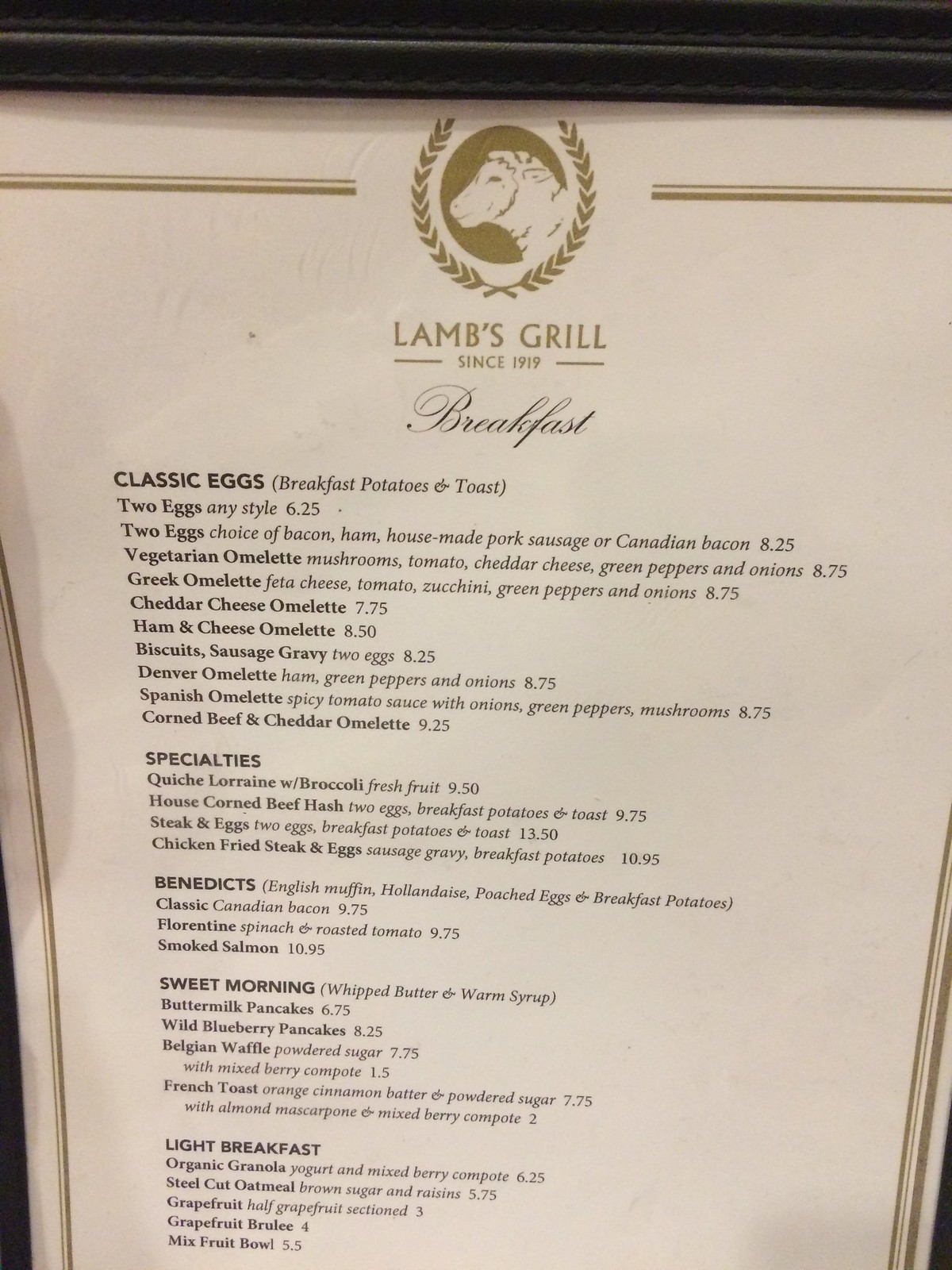The photograph captures a paper menu from a restaurant named "Lamb's Grill," established in 1919. At the top of the menu, there's a logo featuring a lamb encircled by what appear to be leaves or stalks of wheat. The menu is segmented into several sections: 

- "Classic Eggs," offering a variety of egg dishes.
- "Specialties," which includes unique breakfast items with brief descriptions and their respective prices.
- "Benedict's," a section dedicated to different styles of eggs Benedict.
- "Sweet Mornings," listing options such as French toast, pancakes, and waffles.
- At the bottom, the "Light Breakfast" section focuses on healthier choices, including organic granola, oatmeal, grapefruit, and other fruit items.

The detailed layout and diverse offerings suggest a well-rounded breakfast selection catering to various tastes and preferences.